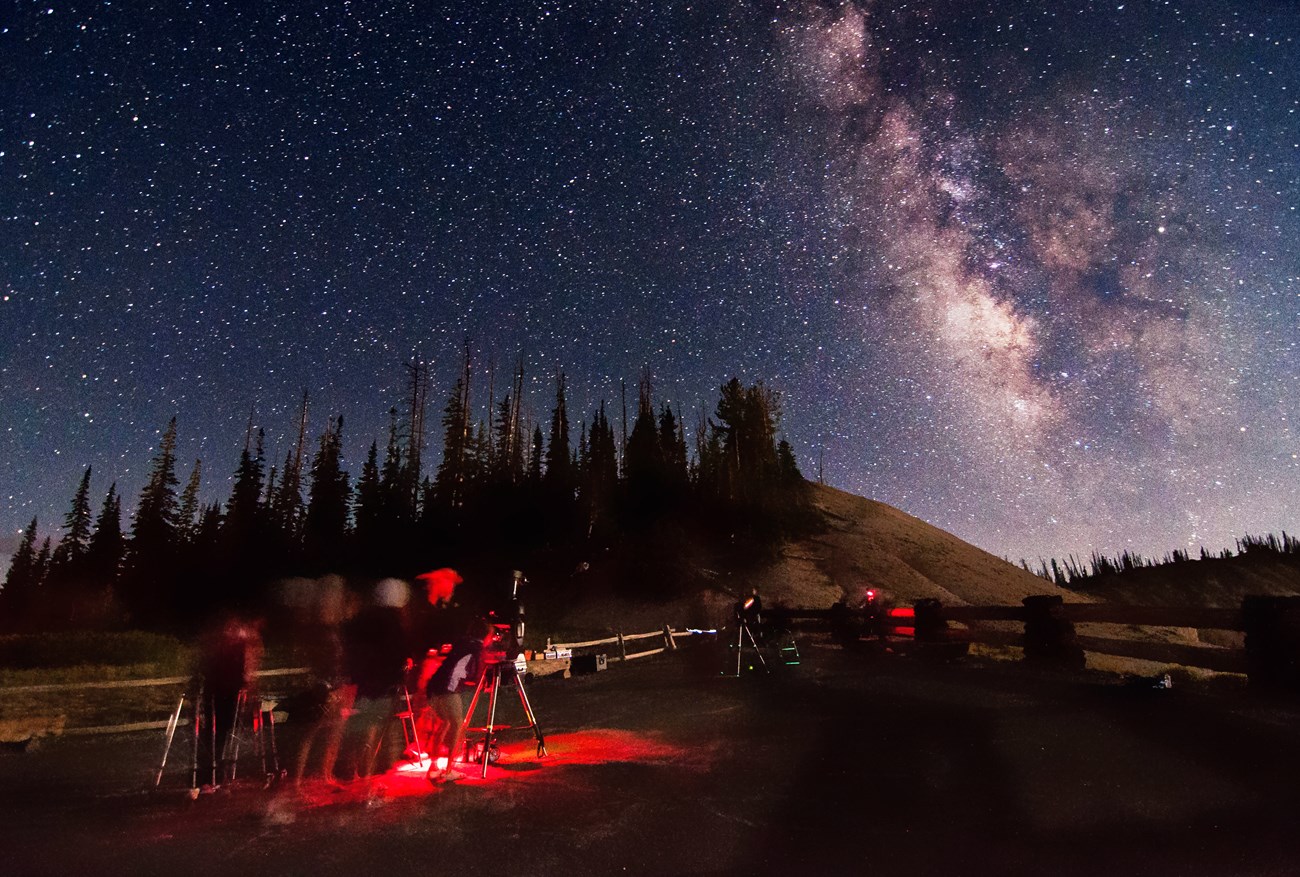The image captures an outdoor nighttime scene featuring a group of blurry figures positioned towards the left side, who appear to be working with equipment resembling microphones or telescopes. This group is illuminated by a red light, which casts a glow on the ground beneath them. In the foreground, directly in front of the people, another device radiates a yellow light, while a similar red light source illuminates the scene from the background. The entire area is enclosed by a fence, beyond which fields and a tree-covered hill are visible. The sky above is filled with numerous stars and showcases the Milky Way, with parts of the sky tinged in a light purple hue. On the right, there is a visible dust-like light in the sky. The image is vibrant and clear, despite the distortion of the human figures, capturing the tranquil night setting with excellent clarity.